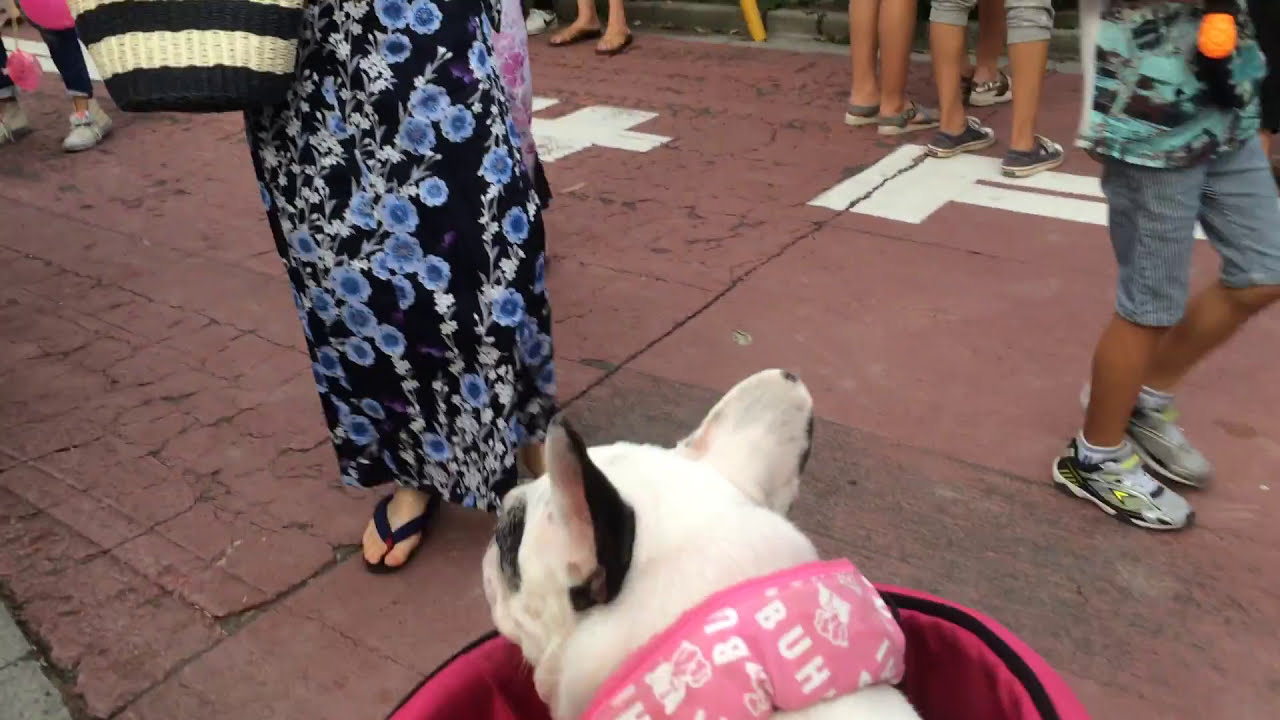In this outdoor image, taken at ground level, the central focus is a black and white dog with a pink collar, seated in a pink and black stroller. The scene is set on a worn, reddish sidewalk with white lines and noticeable cracks. We predominantly see people’s legs and feet, as the image is cut off at the waist for most. Notably, there is a woman in a long, black dress adorned with blue and white floral designs, wearing sandals and carrying a black and tan wicker basket. To the right, a person is walking in blue tennis shoes, gray shorts, and a shirt. The background reveals several people's legs, suggesting a gathering or busy area. The photograph provides a dog’s eye view of the scene, focusing on the dog and giving a glimpse into the various pedestrians around.